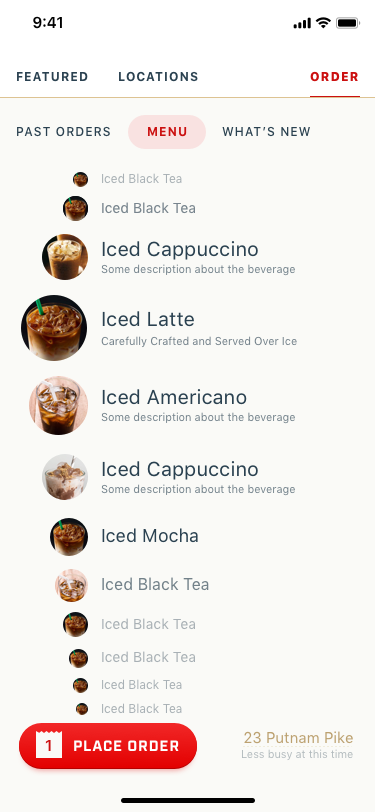This is a detailed screenshot of a coffee place menu from a phone display. The backdrop is white, and in the upper left-hand corner, the time "9:41" is displayed in black. There is a space, and on the right-hand side, the phone signal strength is shown with four bars, followed by icons indicating Bluetooth, Wi-Fi strength, and a black battery symbol.

Below the time and status icons, the menu begins. In the left-hand corner, the word "Featured" appears in black. To the right of "Featured" is "Locations", also in black. A small space separates this from the word "Order" in red on the right-hand side. Underneath "Order" is "Past Orders" in black, and centrally positioned in red is the word "Menu", which is encircled by a light pink bar. To the right of "Menu" in black, it reads "What's New".

The menu items are visually represented with images:
- Towards the center, a small black circle containing an image of a glass of iced coffee is labeled "Iced Black Tea".
- Beneath it, a larger version of the same circle contains the same image, paired with a larger text that says "Iced Black Tea".
- Another circle below shows a glass of iced coffee with white foam at the top; to its right, it reads "Iced Cappuccino", accompanied by a brief description beneath it.
- Following this, a glass of iced coffee with a green straw on the left, white at the bottom, and brown at the top appears; to its right, it says "Iced Latte", with the description "Carefully Crafted and Served Over Ice".
- Next, an iced coffee with a white straw on the left is labeled "Iced Americano" with a descriptive note below.
- Another iced coffee image with a white swirl inside shows up next, marked as "Iced Cappuccino" with an accompanying description.
- A picture of coffee with a green straw on the left-hand side follows, labeled "Iced Mocha" next to a descriptive note.
- Smaller circles follow, repeating the image of iced coffee, marked as "Iced Black Coffee".

The menu continues with decreasing circle sizes, each showing the same glass of iced coffee labeled "Iced Black Tea", which gets smaller and smaller as they descend, repeated four times.

At the bottom of the page is a prominent red bar. In the right-hand corner of this bar is an icon of a white piece of paper with a red number "1" inside it. Next to this icon, in white text, it says "Place Order". To the right, in light brown lettering, it reads "2-3 Putnam Pipe", and underneath, in black, it notes "Less Busy At This Time".